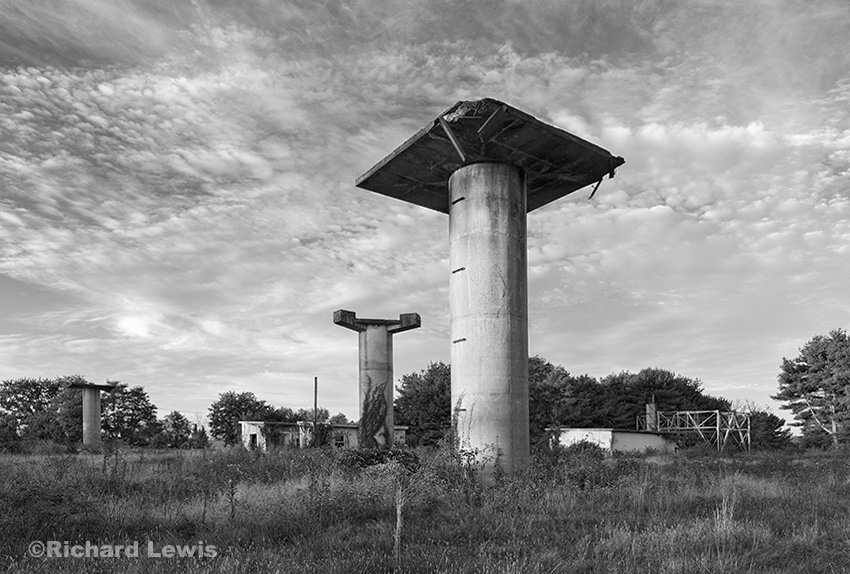This striking black and white photograph, taken by Richard Lewis and bearing his watermark in the bottom left corner, depicts a desolate and seemingly abandoned Midwestern farm landscape under a cloud-speckled sky. Dominating the scene are two prominent cylindrical structures, likely silos or pylons, rising from unkempt grass. In the foreground, the closer silo features a conspicuous square structure perched atop it. Behind it, the second silo has a long, indistinct object protruding from its top. This secondary structure is entwined with climbing vines, adding a touch of nature's reclaiming force. The background reveals an abandoned building, hinting at past activity, and a subtle tree line meets the horizon, completing this evocative portrayal of decay and nature's encroachment.